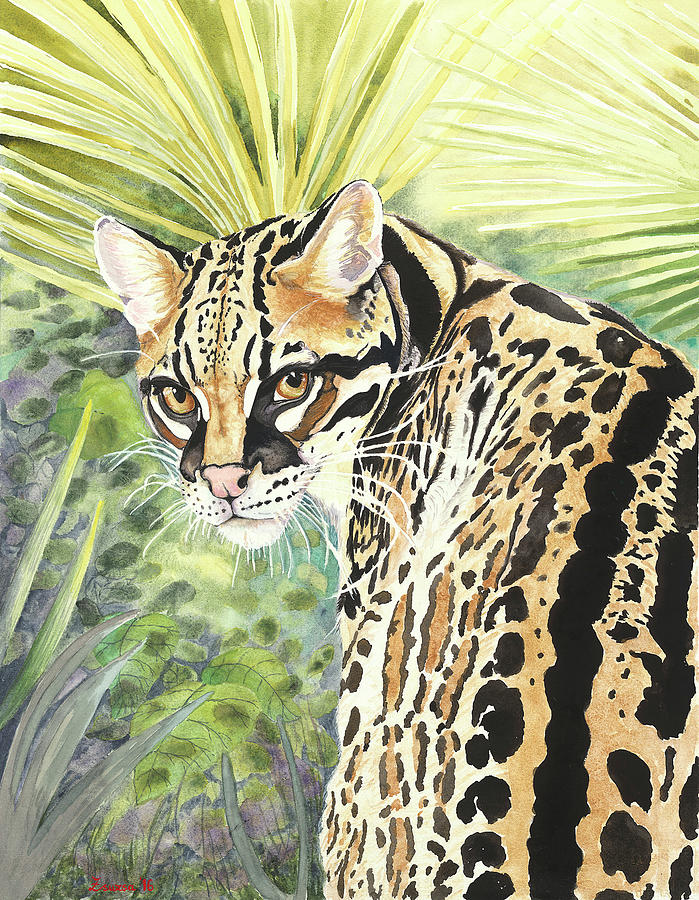This image depicts a detailed and vibrant painting of a large wild cat, possibly a leopard or a jaguar, but some details might suggest it could also be an ocelot or a cheetah. The cat's fur features a striking pattern of tan, black, brown, and cream spots and stripes. It has yellow eyes with dark centers, a pink nose, small triangular ears pointing up, and prominent white whiskers protruding from its closed mouth. The cat's body faces away from the viewer, but it has turned its head back to look directly at us with an intense gaze. The background is lush with green foliage, resembling a dense jungle setting, including palm fronds, ferns, and other leafy vegetation. The backdrop appears to be painted with a watercolor-like technique, and there are visible pencil lines detailing the leaves. Additionally, there is a subtle play of sunshine filtering through the foliage, indicating a sunny day. The painting is signed at the bottom, though the signature is somewhat illegible, possibly reading "Zuzesca 16".